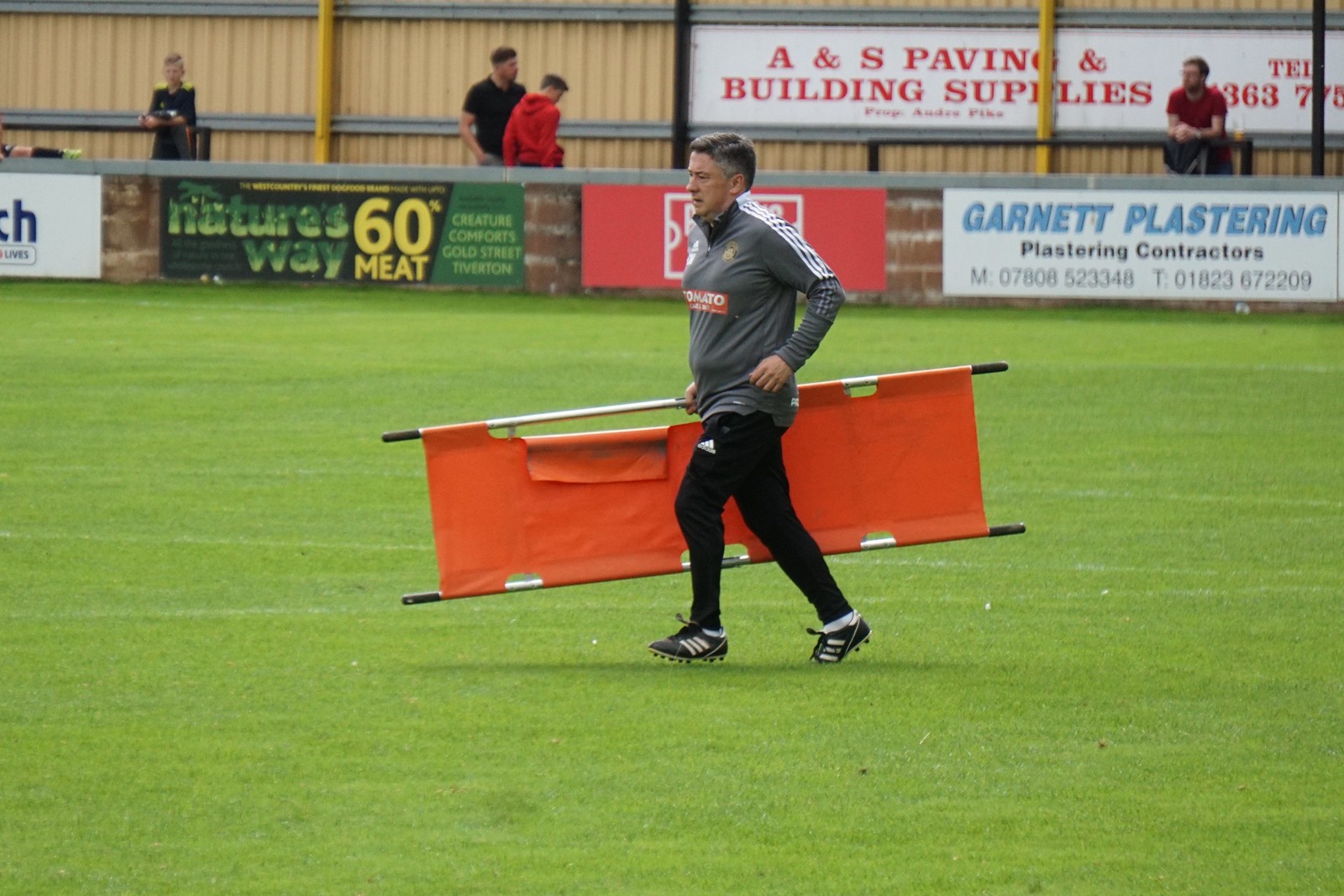The image depicts a middle-aged man on a soccer field, walking leftward with a red stretcher in his right hand. He is outfitted in cleats, black Adidas pants, and a gray jacket adorned with three white stripes down the sleeves and a red logo at the center. The well-manicured green grass of the field contrasts with the advertisements lining the edge, which include sponsors such as Nature's Way, 60% Meat, Garnet Plastering, and ANS Paving and Building Supplies. Beyond the ads, a yellow corrugated metal structure serves as a backdrop, with a few spectators standing and observing the field action. The scene creates a vivid impression of a ready and expectant soccer environment.